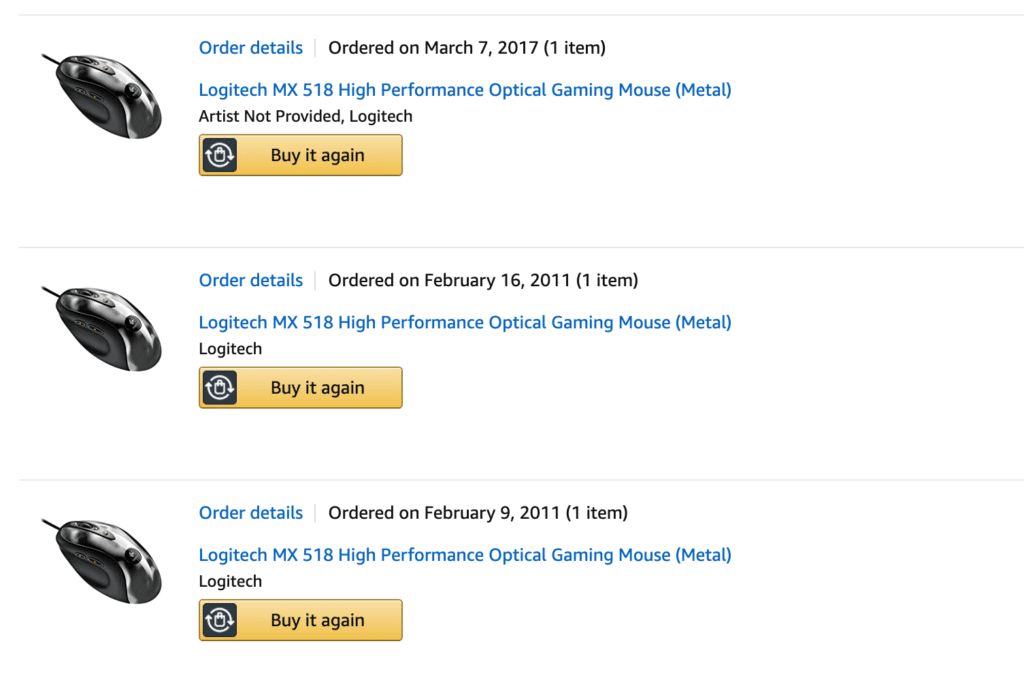The image showcases a slightly wider-than-tall screenshot of three Amazon listings for wired mice, all displayed in consecutive order. Each listing features a consistent photograph on the left side, depicting a gray Logitech mouse with black side pads and a central scroll wheel. The Logitech logo is prominently displayed in the center of the mouse, and a visible cord extends to the upper left direction. 

Each listing is separated by gray horizontal bars and contains specific order details. The first listing indicates an order date of March 7th, 2017, followed by "1 item". The second listing is dated February 16th, 2011, also with "1 item" in parentheses. The third listing shows an order date of February 9th, 2011, similarly noting "1 item".

Below these dates, the product description, "Logitech MX518 high-performance optical gaming mouse," appears consistently across all listings. This text is hyperlinked and includes "(Metal)" in parentheses. The first listing has an additional attribution, "Artist not provided, Logitech," whereas the remaining two listings simply state "Logitech". Each listing concludes with a "Buy it again" button, enhancing the convenience for potential repurchases.